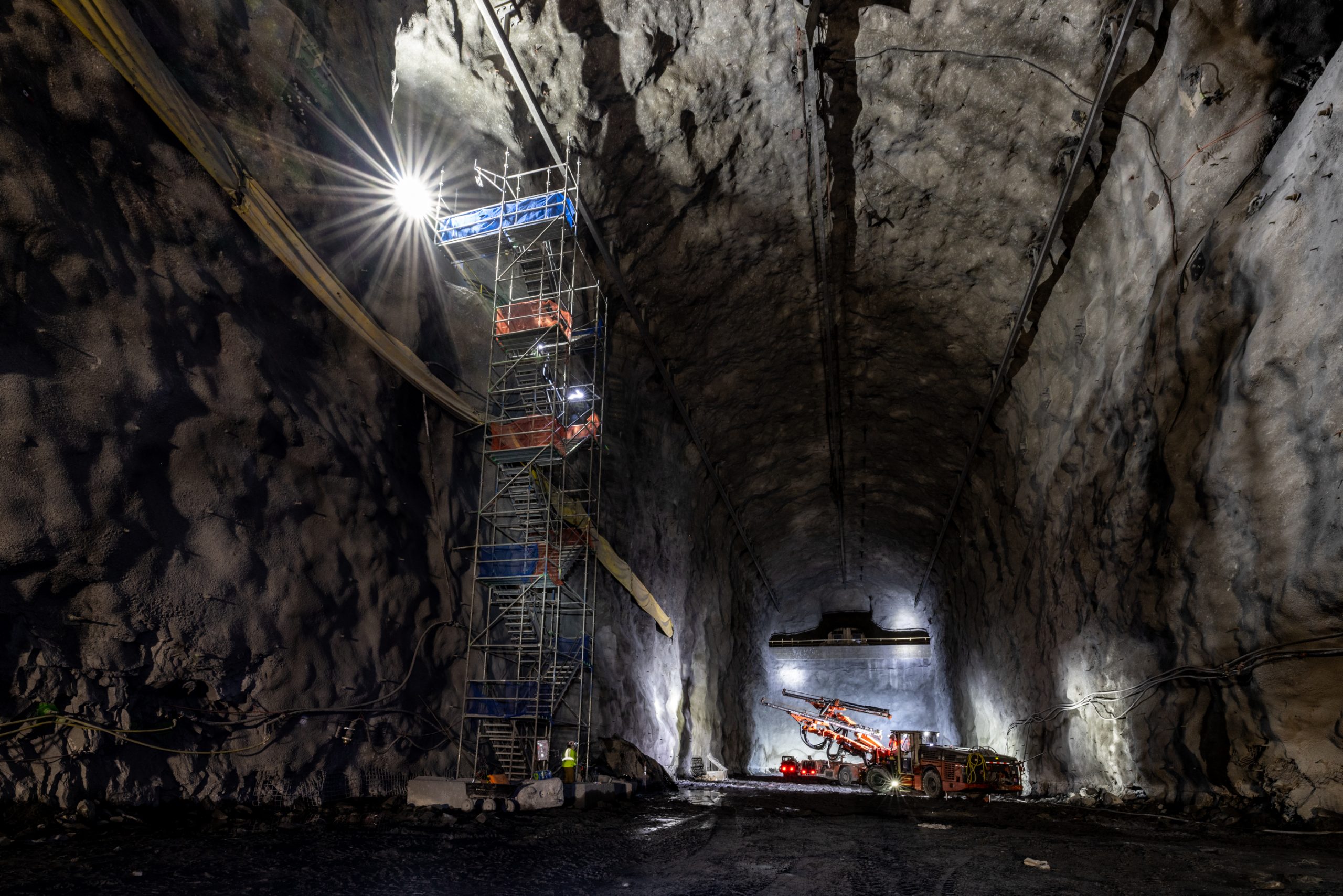The illustration depicts a vast mineshaft or tunnel, primarily composed of dark and light gray rock. The cavern, approximately 50 feet tall and 40 to 50 feet wide, has a large, textured yet smooth interior with metal supports at the top. On the left side, a tall, vertical metal scaffolding extends all the way up to the ceiling, adorned with some piping. At its peak, there's a very bright light emitting star-like rays, casting an ethereal glow.

The foreground shows the ground from a low angle, revealing a dark tar-like floor that extends into the distance. Farther down the hall, the tunnel is more illuminated, showcasing a large excavating truck or vehicle equipped with a bigger light bar above it, brightening the far wall. Overhead, a wire spans the shaft, holding additional lighting fixtures that contribute to the overall visibility within the cavern.